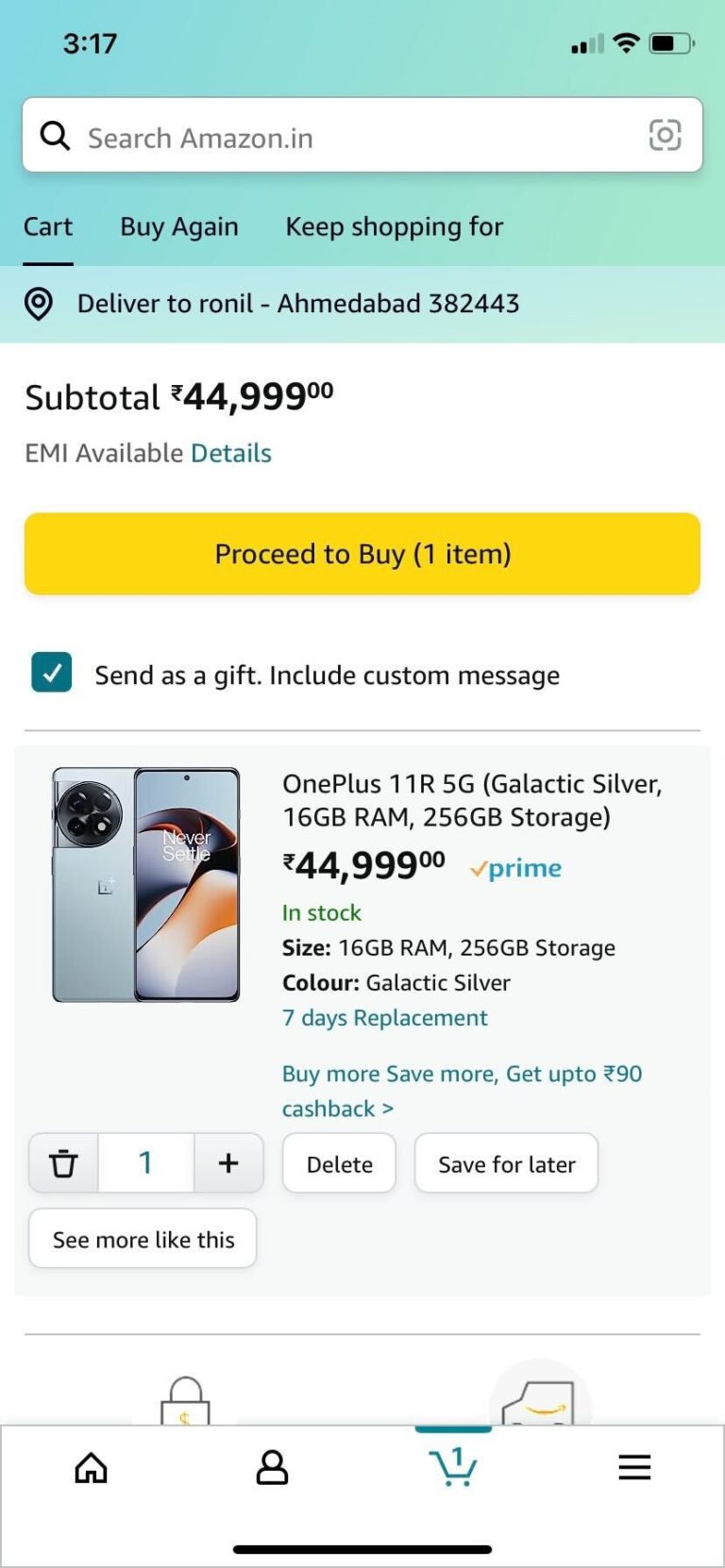**Caption:**

The screenshot illustrates an Amazon.in shopping cart page, as seen on a smartphone screen. The device, connected to Wi-Fi with a battery level at approximately 50%, displays the timestamp of 3:17.

At the top of the page, a gradient pastel green search bar transitions into a slightly darker shade, labeled with "Amazon.in". Below this, navigation tabs, including options such as "Buy Again" and "Keep Shopping For," are visible, along with a cart icon indicating the current viewing tab.

A delivery location is specified: "Deliver to Ronald Ahmedabad 32443." The subtotal displayed is "₹44,999," although a proper currency symbol interpretation was uncertain in the original caption.

An item description occupies the central portion of the screen. The product listed is the "OnePlus 11R 5G Galactic Silver," boasting 16GB RAM and 256GB storage for "₹44,999." The item includes several check marks: "Send as a Gift," "Include Custom Message," and a confirmation of Amazon Prime availability.

The product is in stock with a color option of Galactic Silver and offers a seven-day replacement guarantee. Potential buyers can benefit from up to "₹90 cashback" with certain purchase conditions. Cart management options include adding more items, saving for later, or deleting, with one item currently in the cart.

Finally, the bottom navigation bar showcases icons for "Home," a user profile, and a menu (hamburger icon) for additional options.